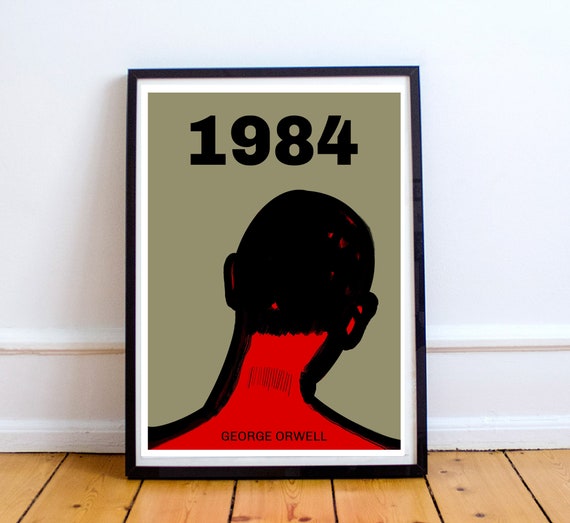The image depicts a framed poster leaning against a white wall with a baseboard, positioned on a wooden floor. The poster features a light olive green background with bold black letters at the top spelling out "1984." Centrally, there is the stylized silhouette of a man's head facing away from the viewer, with short, dark black hair and prominent ears. The man’s skin is painted bright red, and a thin barcode runs across the back of his neck. Below the silhouette, in slightly smaller bold black letters, the name "George Orwell" is inscribed. The black frame of the poster is complemented by a white border that separates the frame from the main image.